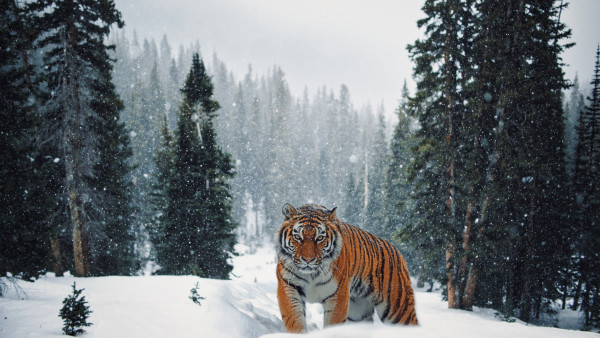In this detailed landscape photo, a majestic tiger stands in the center amidst a snowy forest setting. The tiger, with its striking orange fur adorned with black stripes and a whitish cream underbelly, gazes intensely at the camera, creating a captivating focal point. The animal is positioned slightly to the right, its body angled as if emerging from that side. The ground beneath its powerful paws is blanketed in thick snow. Tall pine trees, their dark green needles dusted with snow, frame the scene on either side, with a small pine tree in the bottom left corner adding to the natural composition. In the background, a dense cluster of pine trees appears muted and slightly blurred, enhancing the depth of the image. The sky above is overcast with gray clouds, contributing to the overall gloomy atmosphere, and delicate snowflakes can be seen falling gently. The combination of the tiger’s vivid colors and the subdued, wintry landscape creates a striking contrast, making the scene both serene and dramatic.